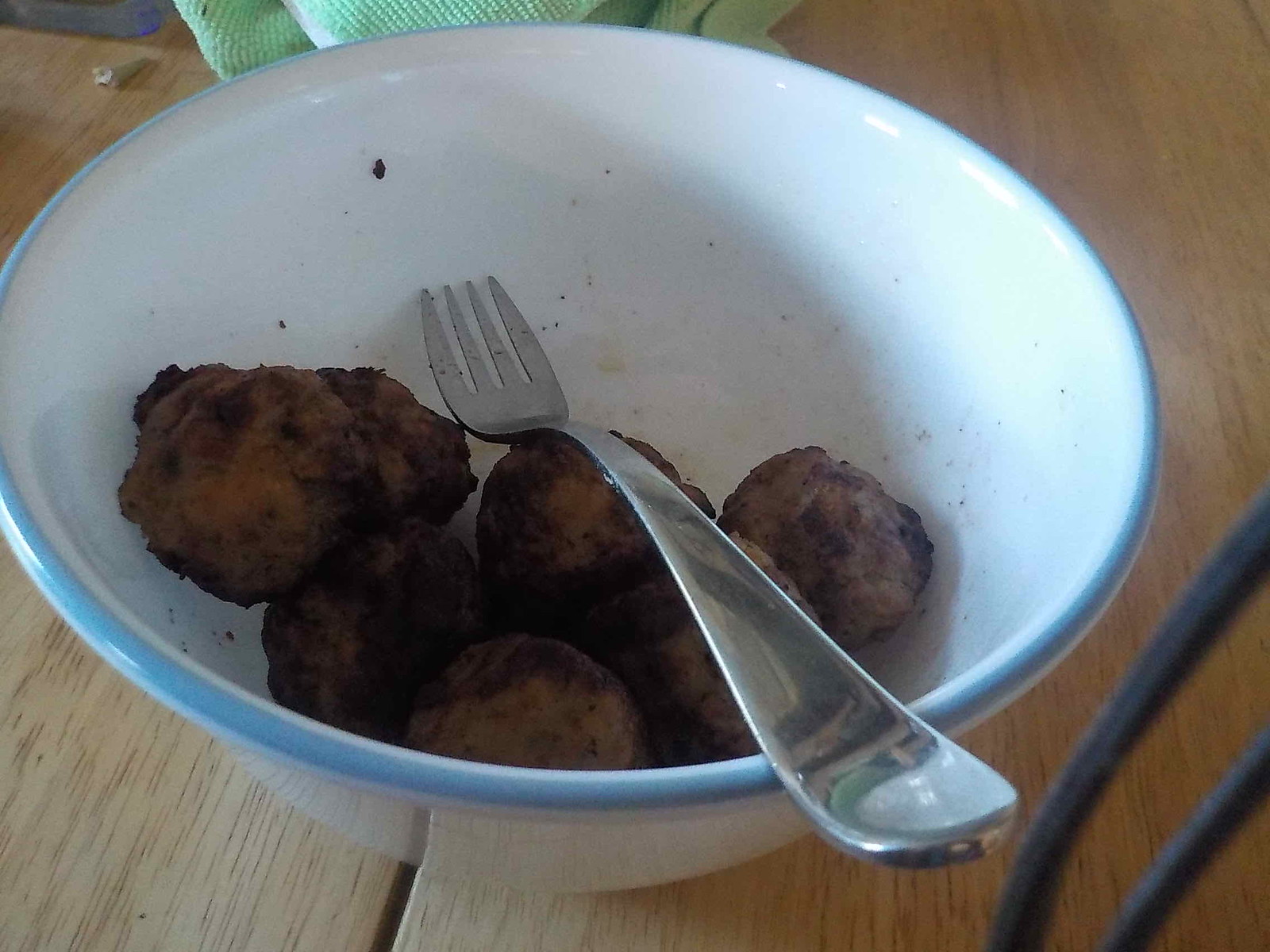In the image, a white enamel bowl with a thin blue rim around the edge sits atop a light brown wood grain table, which showcases a visible split in the pedestal beneath the bowl. Inside the bowl are seven light brown meatballs, each exhibiting a dark, almost blackened fried texture in varying areas, indicating a well-cooked, crispy exterior. A shiny, polished silver fork with four short, closely spaced tines rests on top of the meatballs, its long handle extending outward. To the upper edge of the bowl, a green napkin is slightly visible on the table.